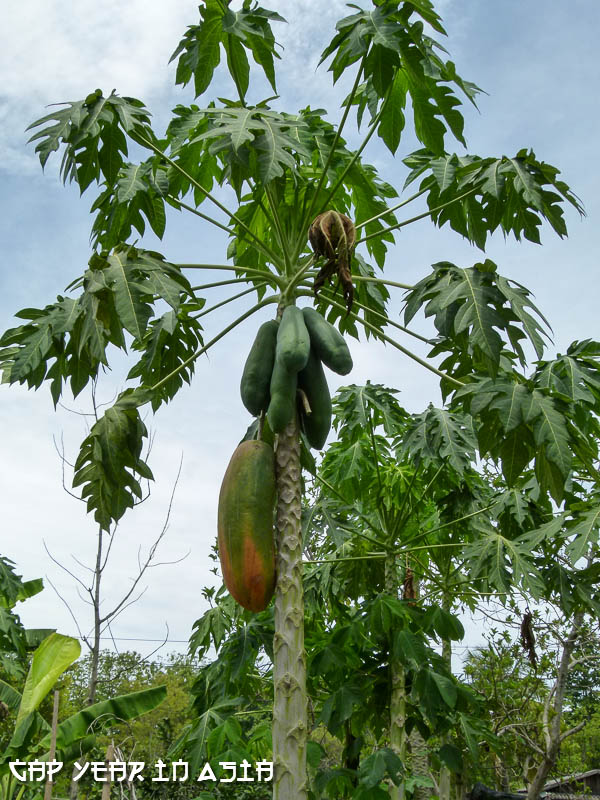This photograph captures a lush and vibrant scene of a tall, slender fruit tree viewed from below, set against a blue sky dotted with white clouds. The tree's thin, light brown-gray trunk extends straight up, supporting long stems that radiate out, ending in thick, wide leaves with jagged, finger-like edges. Prominent in the scene are several large, oblong fruit resembling green eggplants or yams. Most fruits are uniform green, except for one particularly large fruit towards the bottom left, which is a lighter green with an orange-red hue at its base indicating ripeness. The photograph features more greenery and additional similar trees densely packed in the lower third of the image. At the bottom left corner, there is English text styled in Asian lettering, adding another layer of cultural context to the scene.